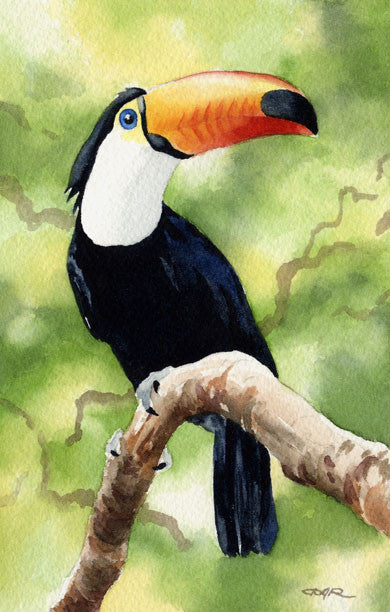The watercolor art print features a vibrant toucan centrally positioned, oriented towards the right on a crooked, tan and brown branch. The toucan sports a substantial orange beak with a black tip and a distinctive black line near the face. Its head displays a notable blend of colors: blue eyes with black pupils, white around the eyes extending to the neck, and a subtle yellow hue behind the eyes. The toucan's body is primarily black, complemented by short, black crest feathers resembling a mohawk. It has gray toes with black claws gripping the branch. The background is a rich medley of green and yellow, interspersed with occasional brown patches. The painting, vertically oriented, bears the artist's signature at the bottom right corner.